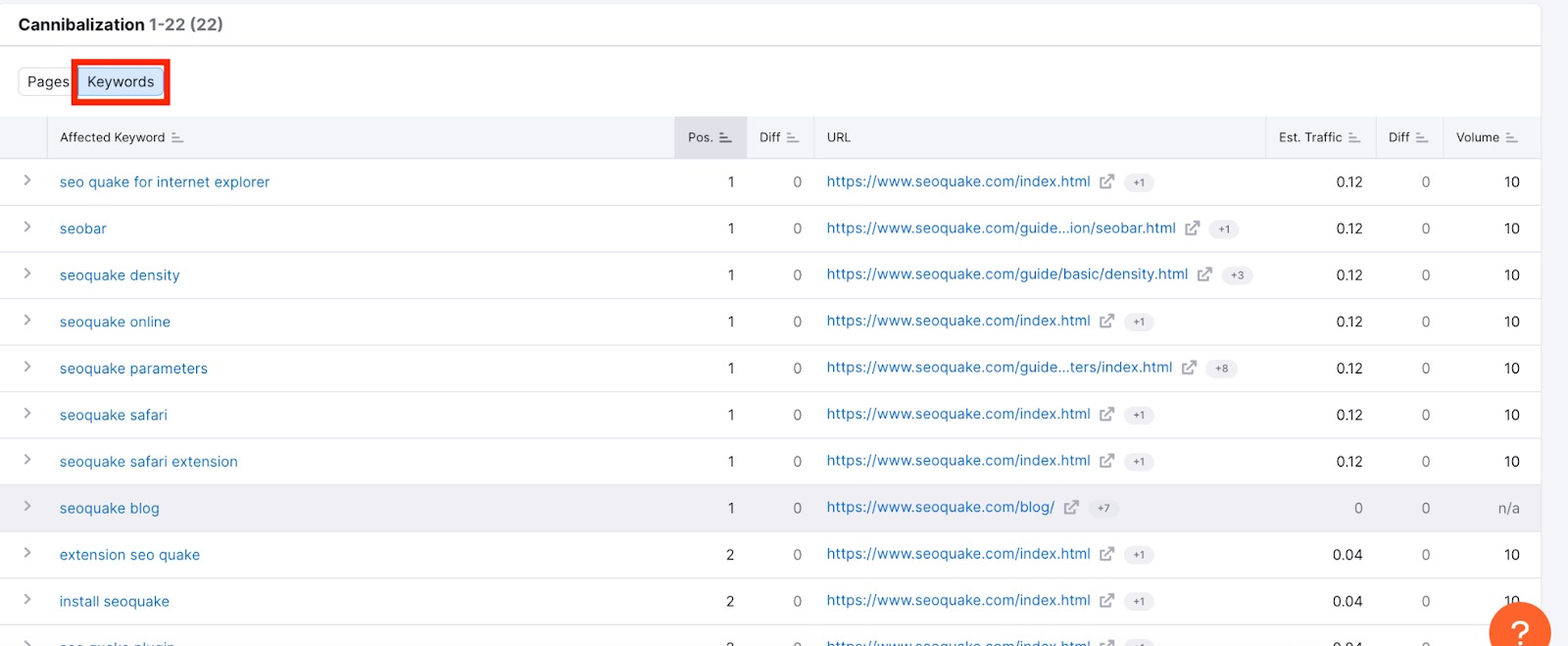This image depicts a webpage titled "Cannibalization 1-22 (22)." Below the title, there are two tags labeled "Pages" and "Keywords," with "Keywords" highlighted by a red box. The top section of the page features a chart header with column titles: "Affected Keyword," "POS," "Diff," "URL," "Estimated Traffic," "Diff," and "Volume." 

The chart contains approximately 10 rows of data. 

In the first row:
- Affected Keyword: "SEOquake for Internet Explorer"
- POS: 1
- Diff: 0
- URL: SEOquake.com/index
- Estimated Traffic: 0.12
- Diff: 0
- Volume: 10

In the second row:
- Affected Keyword: "SEObar"
- POS: 1
- Diff: 0
- URL: SEOquake.com/guide
- Estimated Traffic: 0.12
- Diff: 0
- Volume: 10

At the bottom right of the webpage, an orange question mark icon is visible.